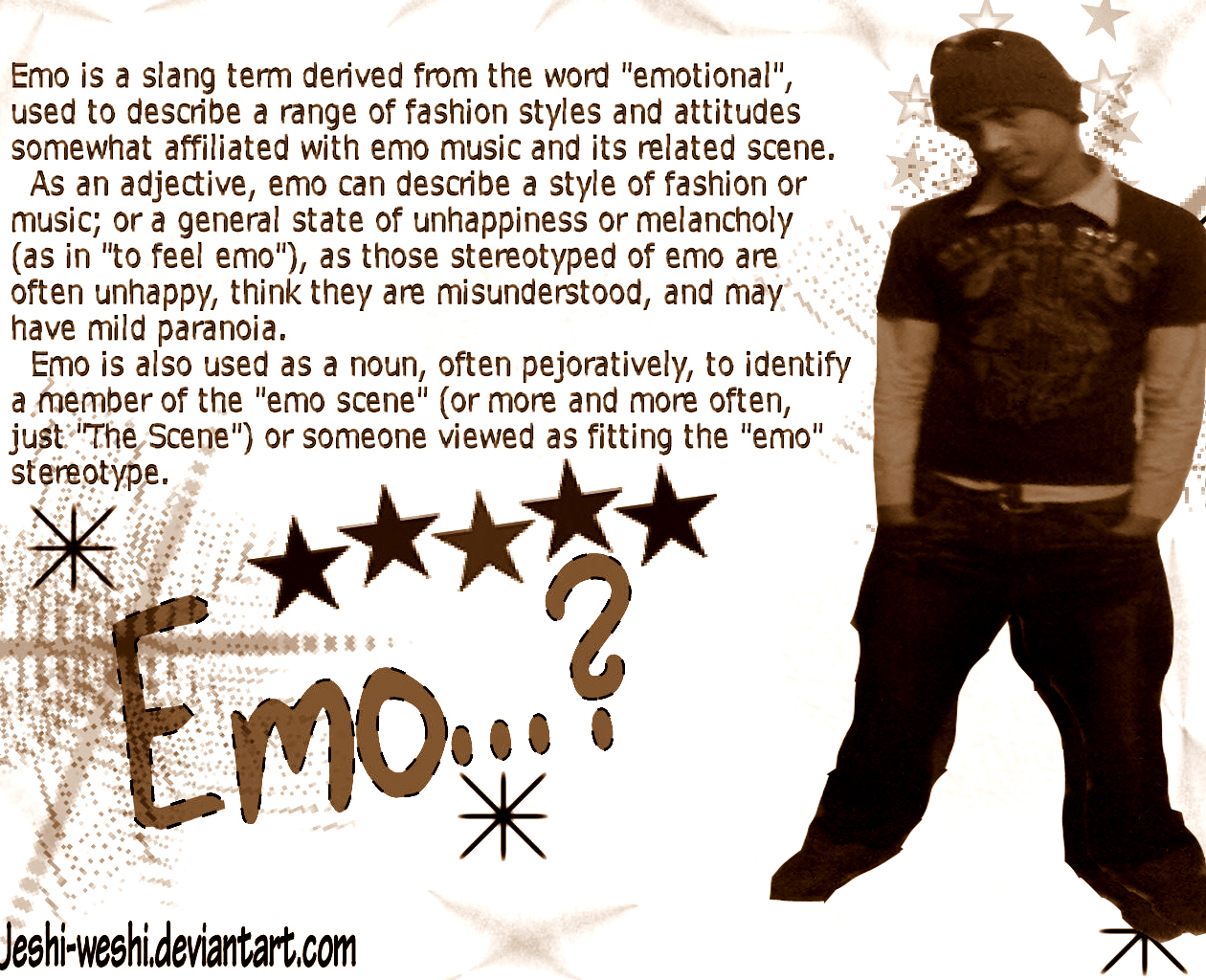In the image, there is a young man standing on the right side, dressed in stereotypical emo fashion: brown pants, a brown shirt with lighter-colored long sleeves underneath, and a cap. His hands are in his pockets and his head is tilted, conveying a contemplative, melancholic demeanor. On the left side of the image, there is text written in brown letters along with five five-pointed stars above. The text describes the word "emo" as a slang term derived from "emotional," used to characterize a fashion style, attitude, and music genre associated with melancholy and a sense of being misunderstood. It notes that "emo" can be used both as an adjective and a noun, often pejoratively, to label someone who fits the emo stereotype. The word "emo?" followed by a question mark is prominently displayed in large brown letters, surrounded by stars. At the bottom left corner, there is a credit to the creator: jessieweshideviantart.com.